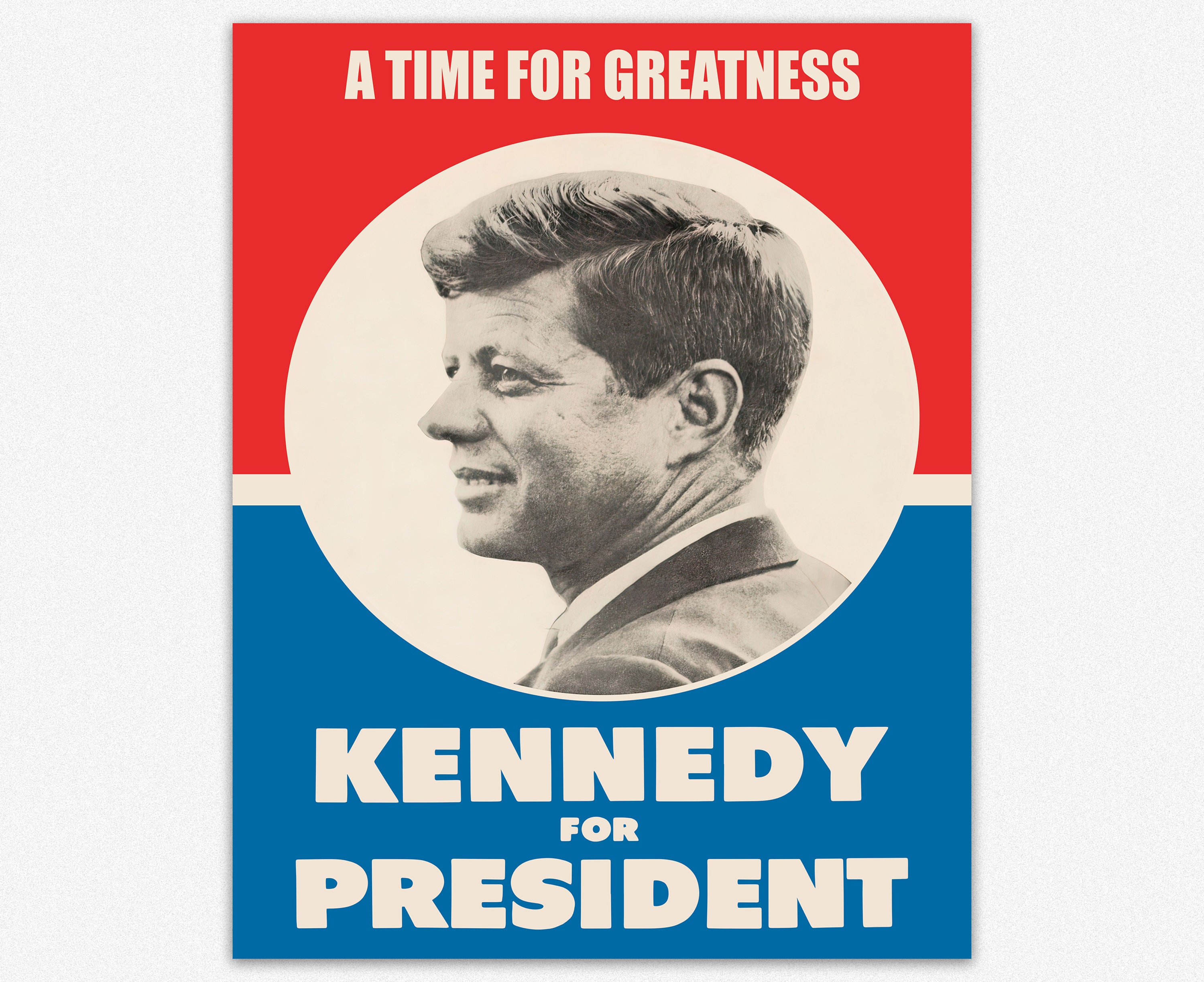The image is a square, light gray in color, featuring a vintage campaign poster for John F. Kennedy in the center. The poster is designed with a red top section and a blue bottom section, separated by a white stripe. In the middle of the poster, an oval frame intersects the white stripe, containing a black-and-white side profile portrait of John F. Kennedy from the shoulders up. His head is turned slightly toward the viewer, revealing his smile and one eye. At the top of the poster, in large white letters, it reads, "A Time for Greatness." The bottom part of the poster has the text, "Kennedy for President," with "Kennedy" and "President" in bold, large white letters, and "for" in smaller white letters. The overall design emphasizes patriotic red, white, and blue colors, and Kennedy's name in large, prominent font, symbolizing the impact and power of his candidacy.